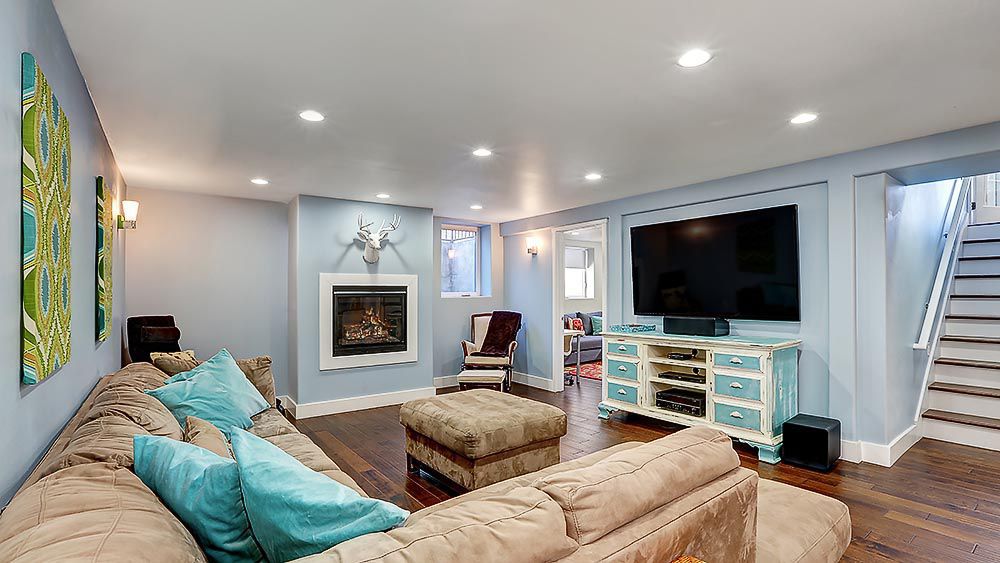The photograph captures a cozy living room with light blue walls and polished dark hardwood floors. The ceiling is painted white and features multiple round recessed lights, all of which are currently illuminated. Dominating the center of the room is a lit fireplace with a white porcelain deer head mounted above it, creating a focal point on the far wall. To the right of the fireplace, a large flat-screen TV is mounted on the wall, above a brown and white TV console. The console is flanked by white stairs with brown wooden steps, leading upwards.

In the bottom left corner of the image, an L-shaped sectional couch in a light tan color is arranged, with a small brown ottoman in front of it. The couch is adorned with green and teal throw pillows, adding a pop of color. On the leftmost part of the couch, two green pillows are visible, and another green pillow is placed on the chaise lounge section on the right end. To the left of the couch, the wall is adorned with a couple of decorative wall hangings. Next to it, a small chair is positioned near a window, bringing in natural light. Adjacent to the chair, there's a doorway leading to another room. Overall, the room has a harmonious blend of light blue and warm brown tones, enhanced by thoughtful details and soft lighting.